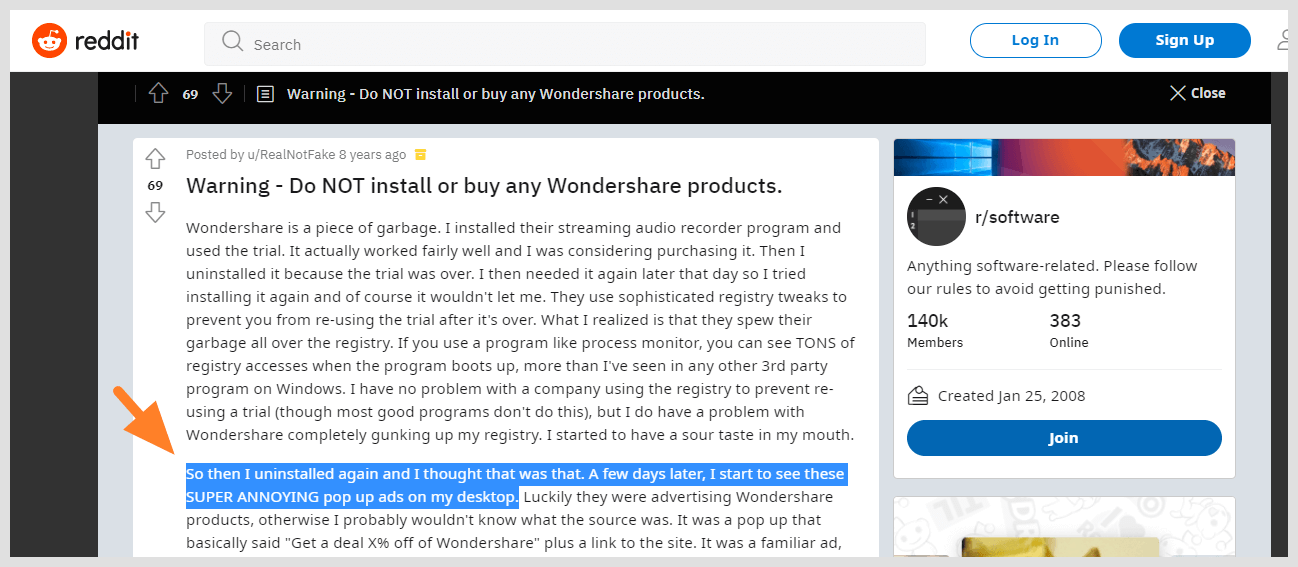This is a detailed screenshot of a Reddit webpage. In the upper left-hand corner, the recognizable Reddit logo—featuring a cartoon alien with red eyes, an antenna on top, set against an orange background—accompanies the word "reddit" in lowercase letters with an orange dot over the 'i'. To the right of this logo is a long, gray rectangular search bar labeled "search." Further to the right, there is an oval "Login" button followed by a blue "Sign Up" oval button.

Beneath this header is a prominent black banner warning readers: "Do not install or buy any Wondershare products." To the left of this banner is a paper icon with a down arrow, along with the number "69" between an up arrow and a down arrow. To the right of the banner is a "Close" button with an 'X' icon. 

Below this setup appears another similar voting section with "69" flanked by an up and down arrow. There is a reiterated warning: "Do not install or buy any Wondershare products." Following this is a lengthy paragraph with a highlighted section in light blue that states: "Then I uninstalled again and I thought that was that. A few days later I start to see these super annoying pop-up ads on my desktop." An orange arrow points to this excerpt.

Further down, there appears to be a boxed section labeled "Our Software," which includes some images and colorful elements in blue and orange, although the details are somewhat indistinct. Below this, it states: "140k members, 383 online," accompanied by a blue "Join" button.